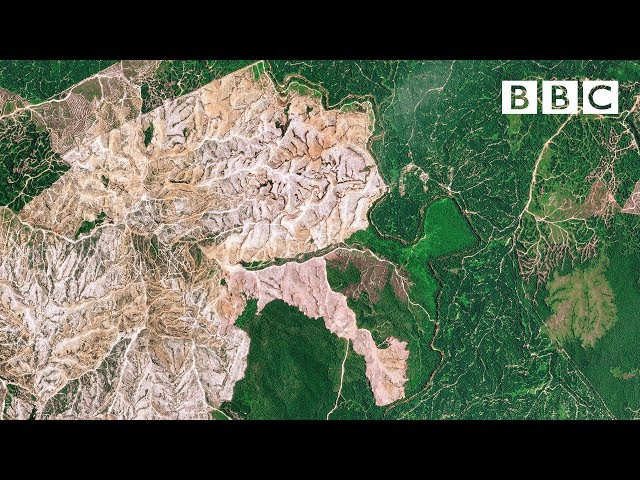The image features an aerial or satellite view showcasing a landscape divided distinctly by color. On the right side, the land is predominantly green, interspersed with white strips and outlines, creating a veiny appearance across the terrain. In contrast, the left side of the image portrays a more barren, desert-like expanse in various shades of beige and brown, with light brown outlines extending from the top to the bottom of the image. These outlines might indicate the presence of mountain ranges or elevated areas. Additionally, the landscape is crisscrossed by numerous wavy lines or trails that cut through the terrain, reminiscent of dirt roads. The top and bottom edges of the image are bordered in black, and situated in the upper right corner within the black border, there is the iconic BBC logo, depicted as white letters on a black background.